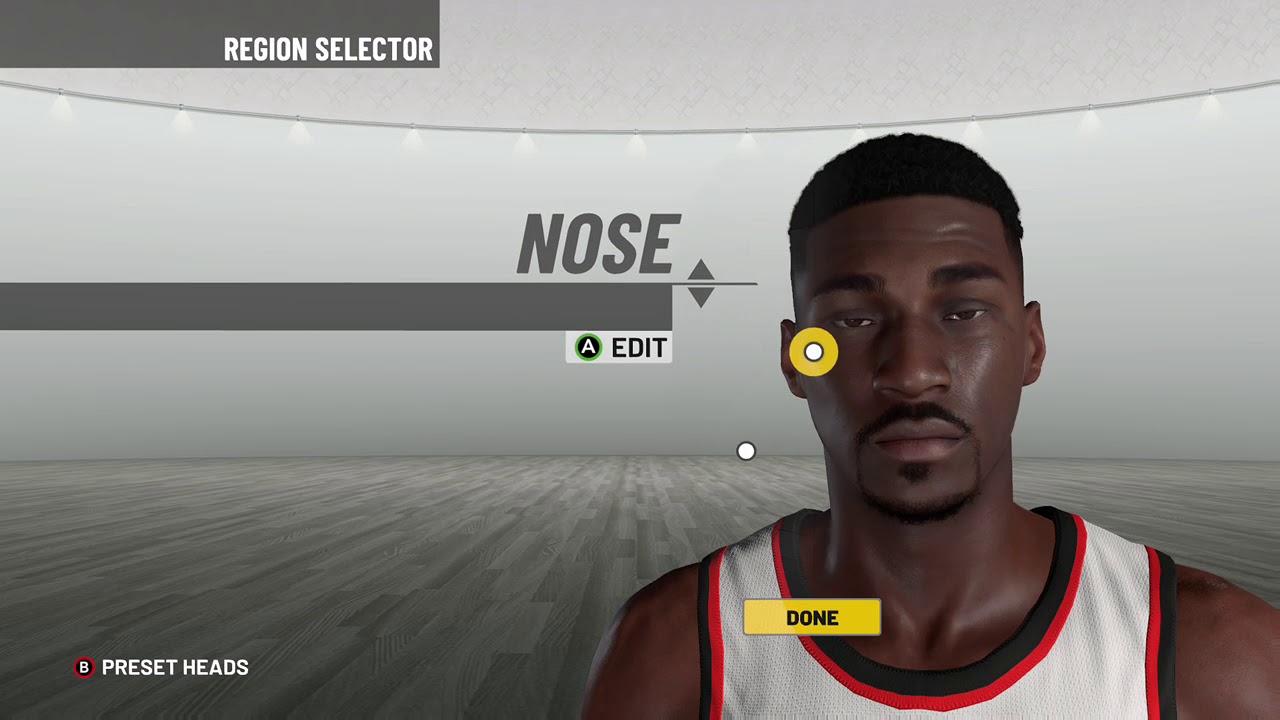A detailed caption for the image could be:

"The rectangular image, oriented horizontally, appears to be a screenshot from a video game, likely during the character creation process. The top left corner features a gray box labeled 'Region Selector.' The background scene is festive with strings of lights draped from the upper left corner, dipping towards the center, and arching back up to the upper right, creating a cozy ambiance. Beneath the lights, a solid gray wall stands, meeting a parquet floor below, which resembles faux wood laminate. In the lower right corner of the image, a black circle with a red outline encloses a white 'B' and is accompanied by the white text 'Set Heads.' Moving back to the left side, another gray box stretches from the left towards the middle. Just above this box, centered, the word 'Nose' is written in gray. Below this, a light gray box with a black circle edged in green contains a white 'A' and the word 'Edit' in black text. To the right of these interface elements stands a character: a Black male figure gazing directly forward, presumably being customized by the player."